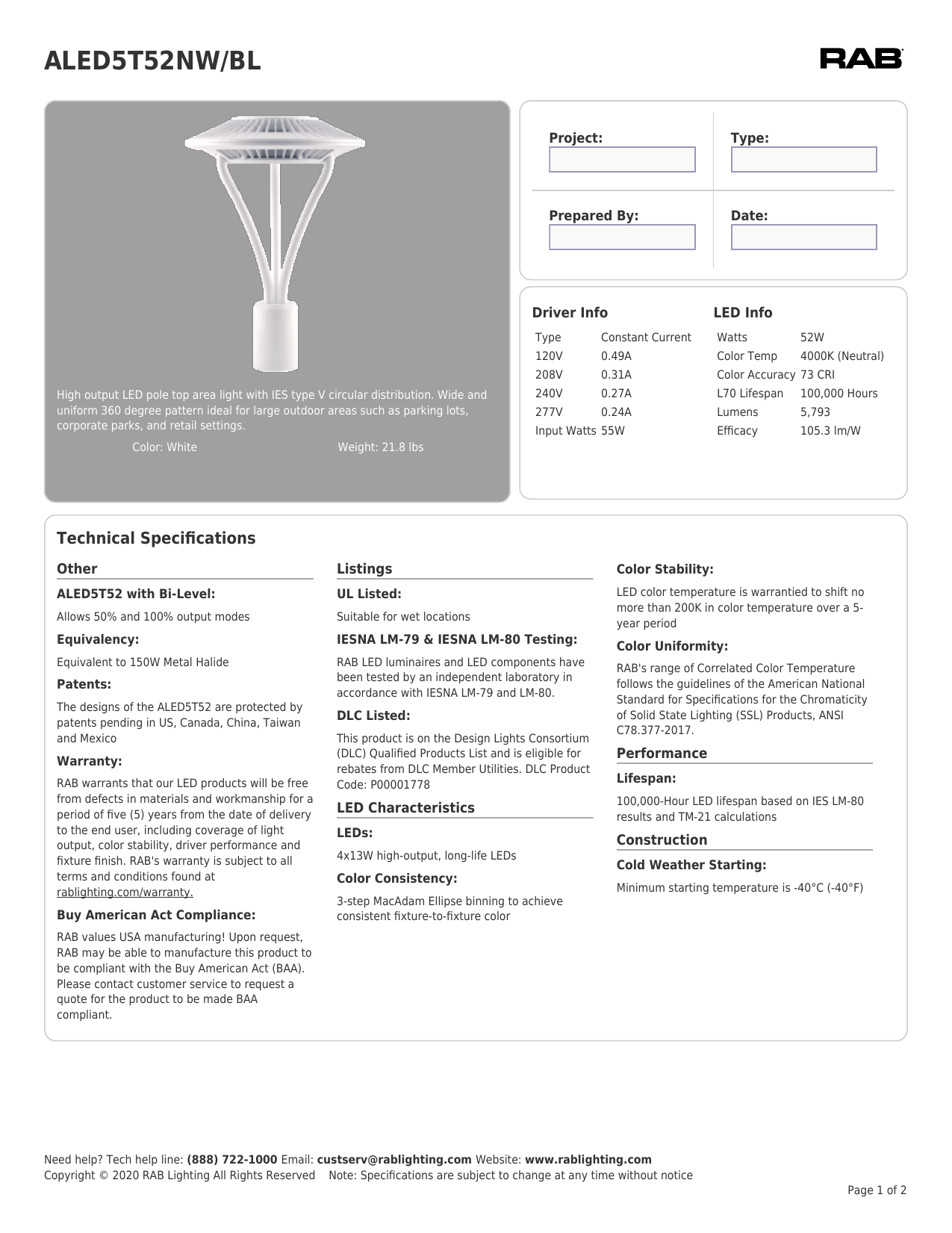**Product Overview for LED Pole Top Area Light (ALED5T52NWBL)**

At the top left corner of the image, the product model "ALED5T52NWBL" is specified, and on the top right corner, the company logo "RAP" is displayed. Below these identifiers, there is a form featuring the fields: "Project Type," "Prepared By," and "Date," allowing users to fill out relevant project details.

Moving downward, detailed product specifications are divided into two categories: "Driver Info" and "LED Info." The "Driver Info" section lists the type as "constant current" with an input wattage of 55 watts. The "LED Info" section specifies an LED wattage of 52 watts and an efficiency rating of 101.3 lm/W.

On the left-hand side of the image, a visual representation of the device is showcased against a grey background, with the device illustrated in white. The accompanying text provides a comprehensive product description:

- **High Output LED Pole Top Area Light**: The device is labeled as an ideal lighting solution for expansive outdoor areas like parking lots, corporate parks, and retail settings. 
- **IES Type V Circular Distribution**: It offers a wide and uniform 360-degree lighting pattern.
- **Color and Weight**: The light is white and weighs 21.8 pounds.
  
Additionally, the **Technical Specifications** section mentions the ARDA feature, which allows for 50% and 100% output modal equivalency comparable to a 250-watt metal halide light. The design of the ALED5T52 is protected by patents pending in the US, Canada, China, Taiwan, and Mexico.

**Warranty Information**:
RIP guarantees that their LED products are free from defects in materials and workmanship for a period of five years, from the date of delivery to the end user. This warranty covers aspects such as light output, color stability, driver performance, and fixture finish, subject to the terms and conditions outlined on redlighting.com.

**Listings and Compliance**:
- **Buy American Act Compliant**
- **Suitable for Wet Locations**
- **DL Listed**

Finally, additional product attributes are listed on the right side, covering "Color Stability," "Color Uniformity," "Performance," and "Construction." The text is in black against a white background. At the bottom right, you can find the pagination indicator: "Page 1 of 2."